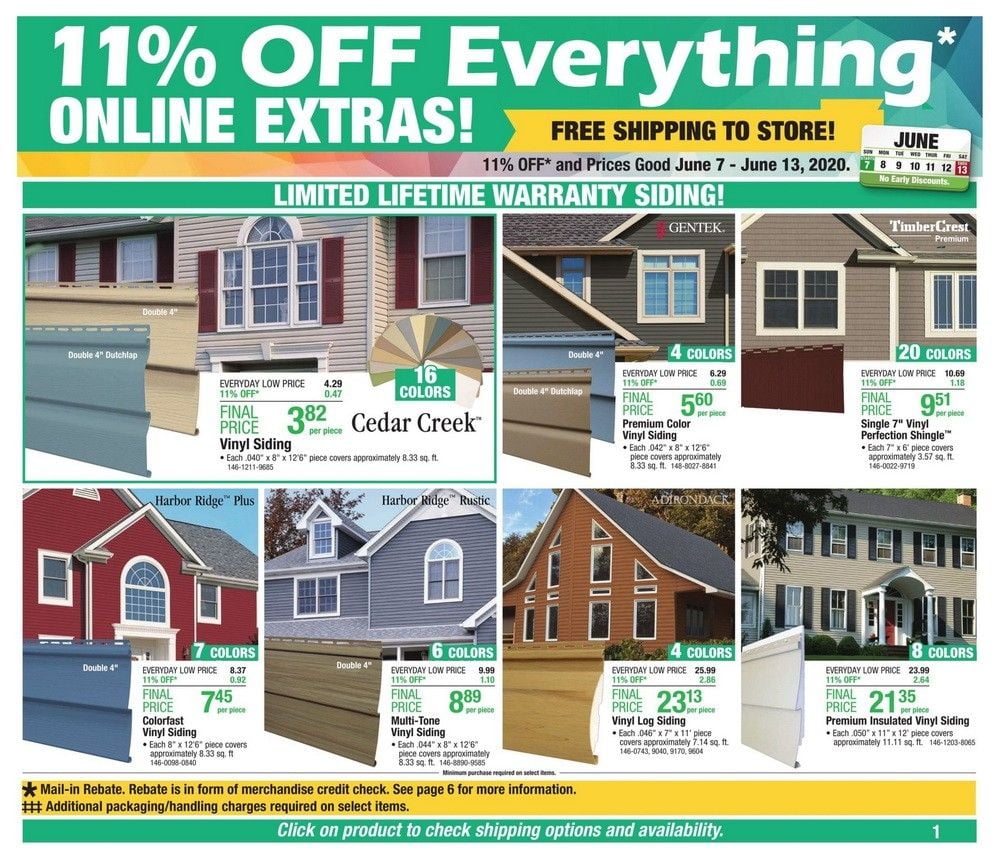This image appears to be an advertisement from Menards, prominently featuring a promotional offer at the top that states, "11% off everything" with an additional note, "online extras." A banner beneath this emphasizes "free shipping to store." Notably, the word "everything" is marked with a small star, indicating that there might be fine print or certain exclusions, although these details are not visible in the image.

In the upper section of the ad, "limited lifetime warranty" is mentioned, suggesting the items come with this warranty. The advertisement focuses on various types of siding, showcasing a range of colors including gray and tan. Specifically, vinyl sidings are highlighted, with one named Cedar Creek priced at $3.82 as the final price. Additional prices for various siding options include $5.60, $7.45, $8.99, $9.51, $21.35, and $23.13.

At the bottom of the ad, there's an instruction to "click on the product to check shipping options and availability." Additionally, a yellow section mentions a mail-in rebate, specifying that the rebate comes in the form of merchandise credit. The notice about the rebate continues in this area, though it's not fully visible in the image.